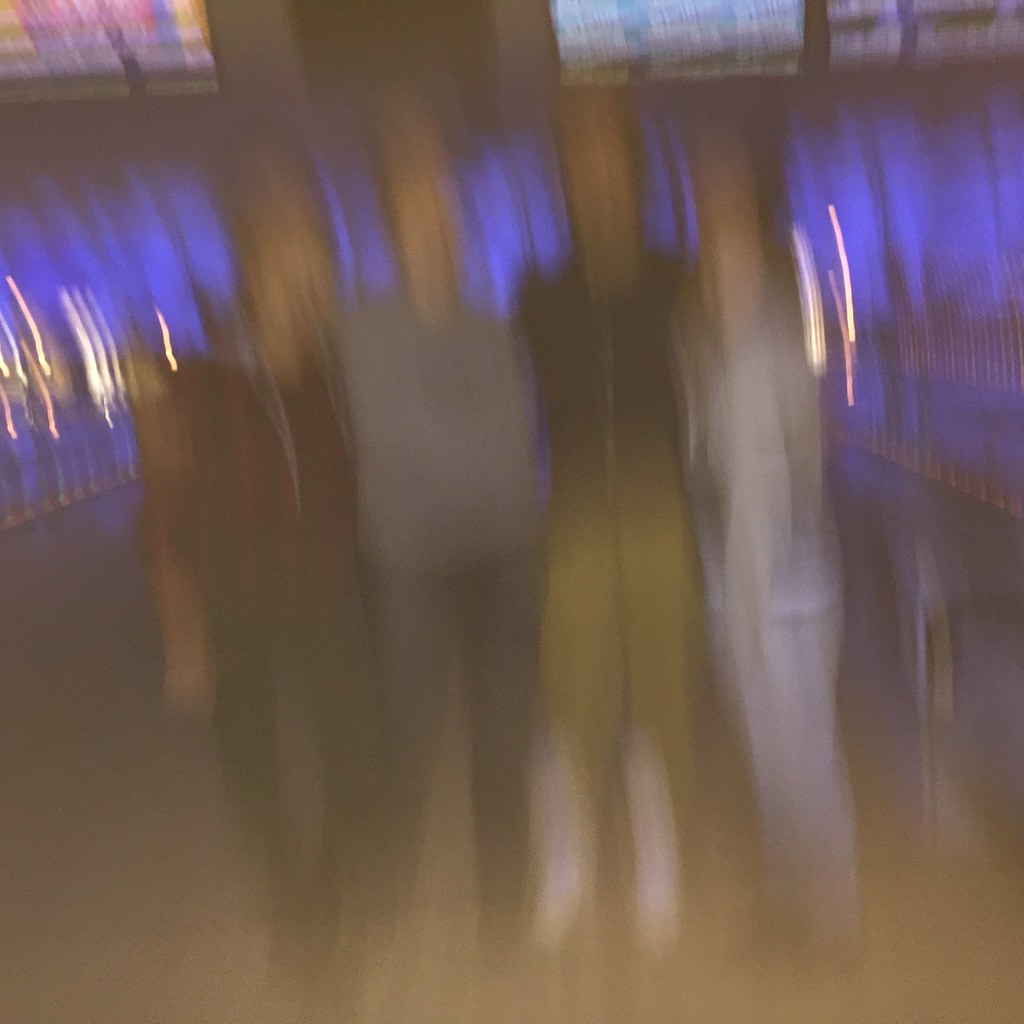In this square image, we see a blurry photograph, seemingly taken indoors. Despite its lack of clarity, certain details can be discerned with some imagination. The scene features a brown floor on which four fair-skinned individuals stand, surrounded by areas illuminated with vibrant lighting. This lighting suggests a setting like a casino, with neon white and blue hues casting a glow on possible rows of slot machines. 

From left to right, here is a detailed description of the individuals:
- The first person on the left is dressed entirely in dark clothing, consisting of a sleeveless shirt and dark pants.
- Next, moving to the right, is an individual in a gray shirt paired with dark pants.
- The third person sports a dark shirt, gold pants, and striking white boots that reach up to their knees.
- The person on the far right is wearing a light long-sleeved shirt or jacket along with light-colored pants.

The blurred quality of the image and the imaginative interpretation of its setting contribute to the mysterious and engaging atmosphere of the photograph.